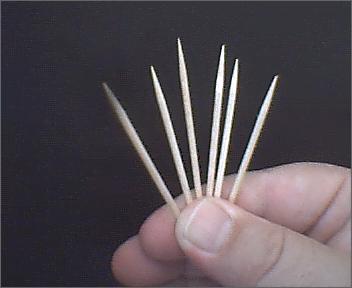A close-up photograph features a fair-complexioned hand against a completely black background. The image zooms in on the person's thumb, index finger, and middle finger, all neatly manicured, as they hold six clean, pointy, wooden toothpicks with a light beige color. The toothpicks are spread apart, held in a fanned-out manner resembling a flower or a deck of cards, with small gaps between each. Only the top parts of the toothpicks are visible as the lower parts are obscured by the fingers.